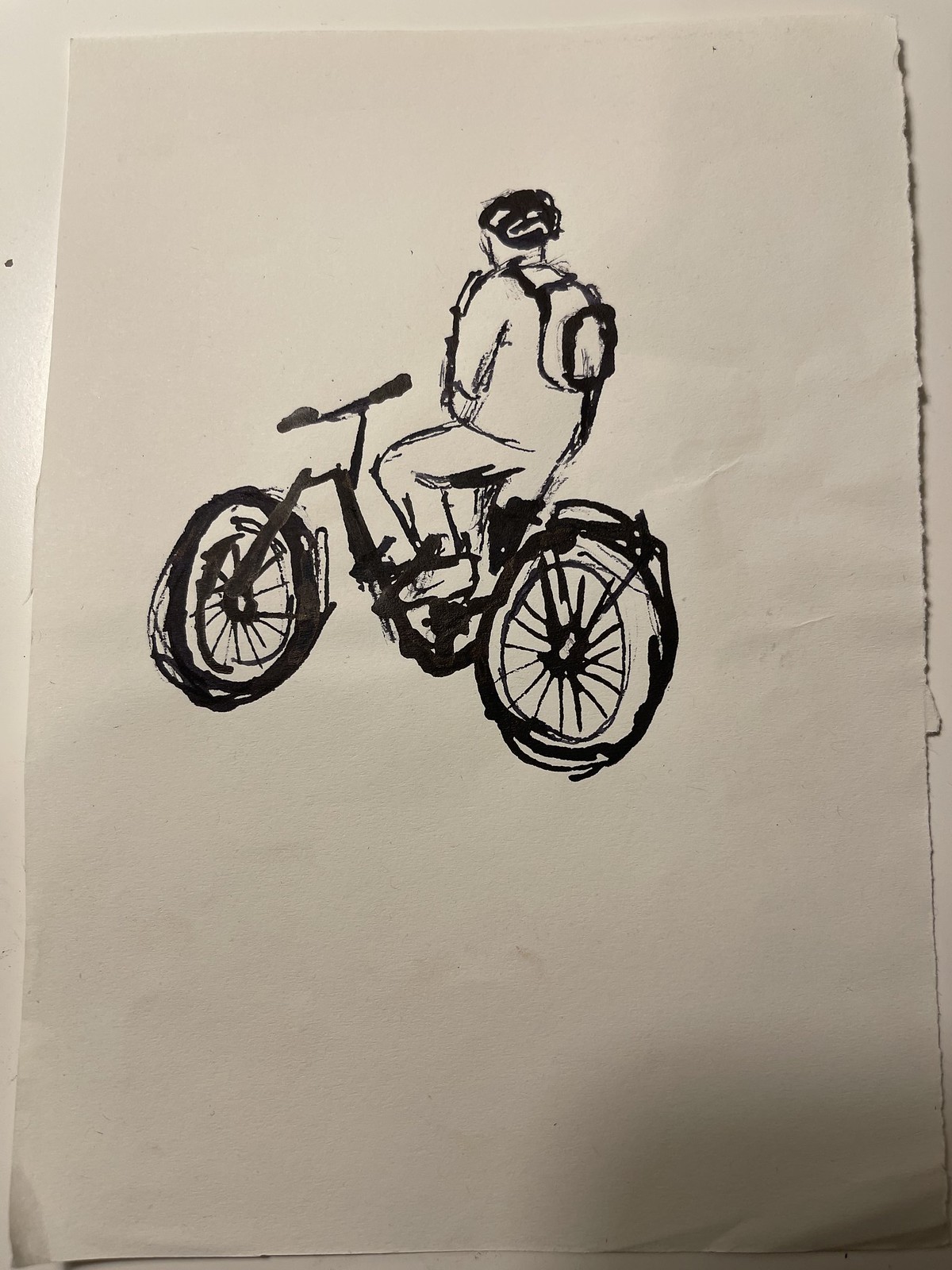This black and white photograph depicts a piece of A4 paper, manually cut and uneven in shape, slightly narrower at the top. There are torn edges on the right side, suggesting it was ripped from a book or artist's notebook. The paper lies on a white table. The drawing, executed in heavy black ink, features a cyclist moving from right to left, viewed from a back-side-left angle. The cyclist, wearing a helmet and a backpack, appears to have black shaded hair and a long sleeve shirt. Notably, their hands are not gripping the low-set handlebars of the bicycle, suggesting a sense of motion or perhaps a daring posture. The overall scene captures a moment of dynamic, yet risky, movement.